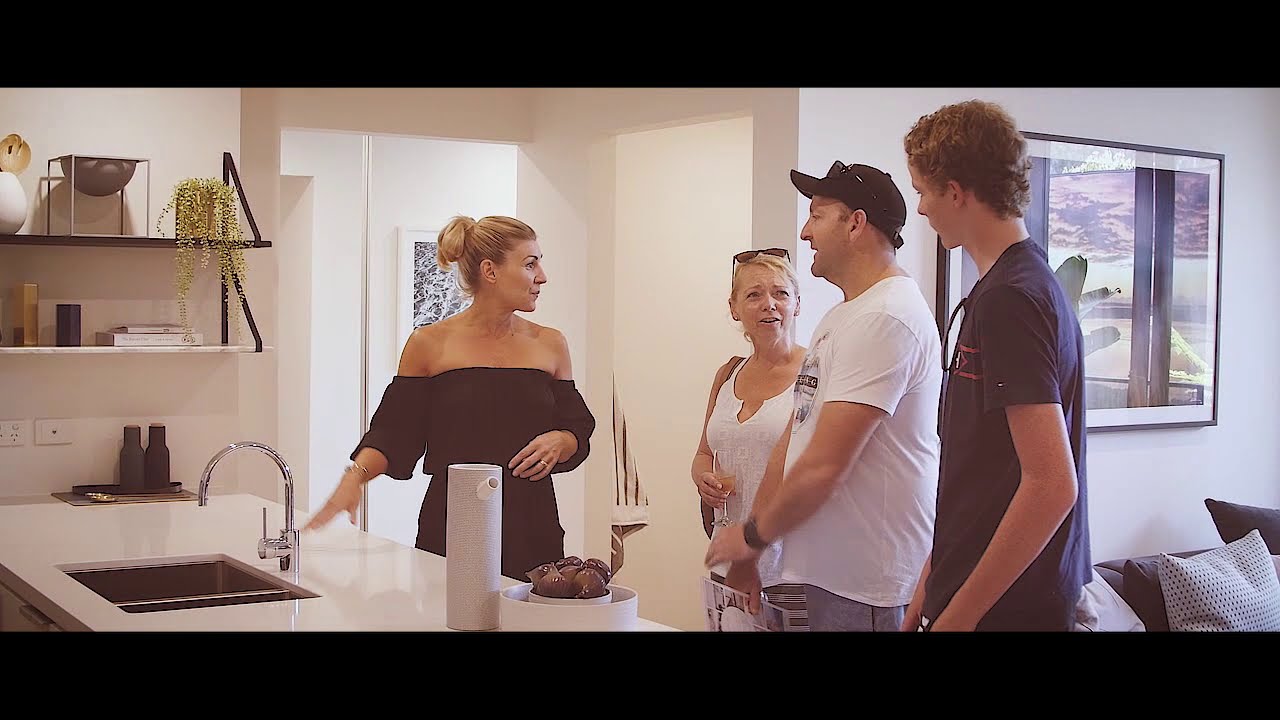The image captures a spacious, brightly-lit interior of a house, where two distinct areas — a kitchen and a living room — blend seamlessly. On the left, the kitchen features a pristine white countertop with a sink and a bowl of fruit, possibly onions, placed prominently. Shelving with books can be seen, along with a clean faucet and a portrait on the wall that is black and white. In the center, a woman in an off-the-shoulder black top stands near the countertop, smiling slightly and gesturing as if explaining something. 

To the right, the living room houses a couch adorned with multiple cushions in shades of grey, white, and black, including some with dots. A large portrait, approximately 40 by 30 inches, hangs on the wall above. Four people are in the scene: a man in a black cap and white t-shirt with sunglasses perched on his collar, and their teenage son, taller than his dad, wearing a dark shirt. Next to them is a second woman in a white tank top with blonde hair in a ponytail and sunglasses on her head, sipping from a wine glass. The bright daylight filtering through the room creates a warm and welcoming atmosphere.